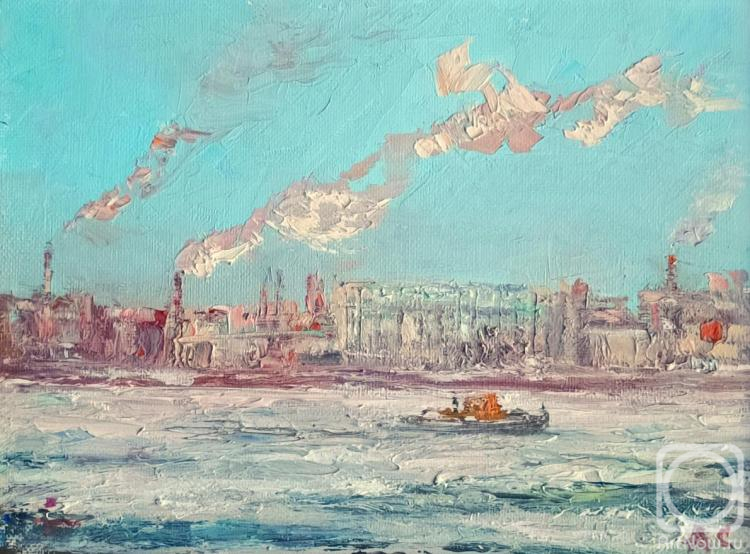This image is a highly textured acrylic painting depicting an industrial cityscape along a shoreline. The canvas texture is notably visible, particularly in the vibrant, light blue sky. The sky is punctuated by clouds of white smoke billowing from factory smokestacks atop several buildings on both the left and right sides of the composition. These factories, rendered in a blend of gray, red, and bluish hues, dominate the scene and give an impressionistic feel, with details purposefully blurred to evoke a sense of haze and pollution.

Below the skyline, a river or ocean, characterized by its swirling white streaks and patches of blue, extends across the lower portion of the painting. Near the center-right, a small boat navigates through the water, moving from left to right. The boat itself is grayish-white with an orangish-red cabin area. A shadowy figure, possibly a person, stands within this boat, adding a human element to the industrial scene.

The painting's texture is rich and voluminous, achieved through layers of gel and thick brushstrokes. Furthermore, in the bottom right corner, there is a watermark featuring a camera outline and partially legible text, seemingly reading "rnow.roo," which adds a modern touch to this evocative industrial depiction.